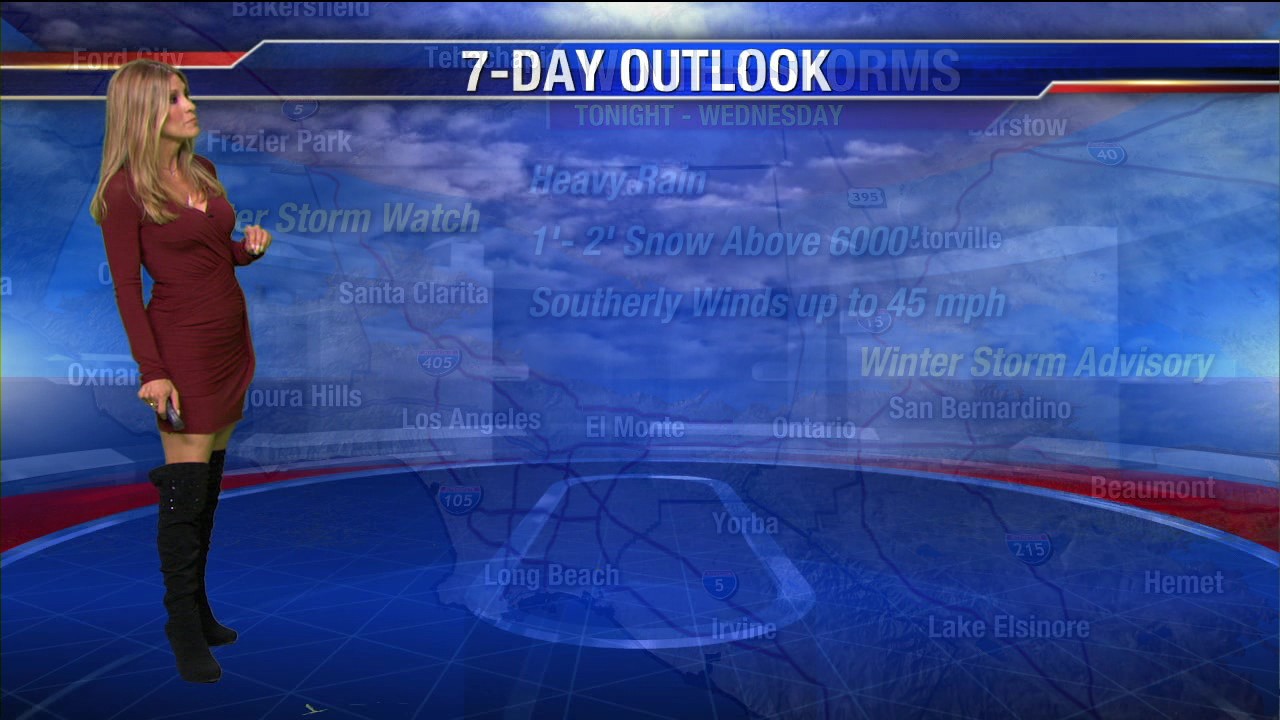The image depicts a weather forecast segment on TV featuring a blonde weathercaster on the left, dressed in a long-sleeve maroon dress and high black boots, with a remote in her right hand. She is looking to her right at the forecast display. The top part of the image has a blue bar with white, all-capital letters reading "SEVEN-DAY OUTLOOK." The background underneath is a light blue with faint clouds and layered text in white and light blue. This includes weather details such as "Winter Storm Watch," with specific forecasts mentioning heavy rain, 1 to 2 inches of snow above 6,000 feet, and southerly winds up to 45 miles per hour. Locations listed include Los Angeles, Long Beach, Santa Clarita, San Bernardino, El Monte, Ontario, Yorba, Irvine, Lake Elsinore, and Hemet, implying the forecast is for California. Additionally, there is a "Winter Storm Advisory" for San Bernardino mentioned at the bottom right. The entire display combines sans-serif fonts, some italicized text, red graphic elements, and thin gold lines, creating a dynamic visual presentation.